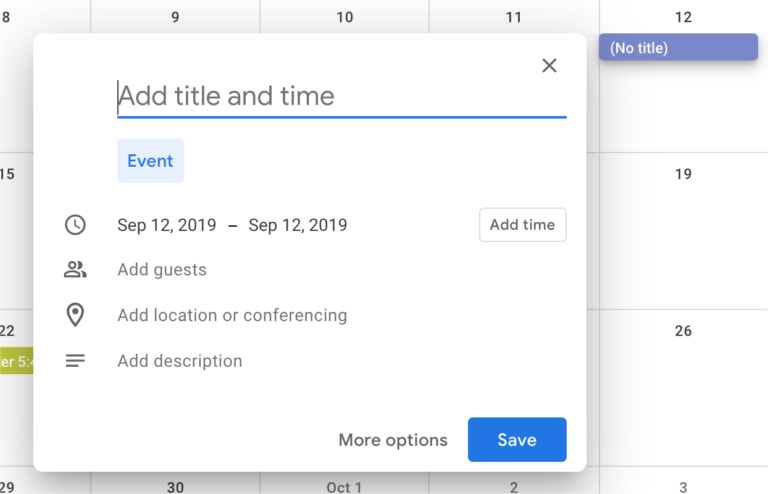In this image, someone is actively creating an event on a digital calendar interface. The background prominently features a calendar with the date September 12th highlighted, indicating the day for which the event is being scheduled. The central focus is on a pop-up menu where the individual is inputting event details.

At the top of the menu, there is a text box labeled "Add title and time," inviting the user to provide a name and timing for the event. Directly below, the word "Event" is displayed, signifying the type of entry being created. This is followed by the specific date range for the event, reading "September 12th, 2019 through September 12th, 2019," which emphasizes that it is a single-day event. Adjacent to this date range is an option to "Add time," allowing the user to specify the exact timings.

Further down, there are several additional fields: "Add guests," for inviting participants; "Add location or conferencing," for specifying a physical location or virtual meeting details; and "Add description," for providing any further information about the event. At the bottom of the pop-up menu, there is a button labeled "More options" for additional customization. Finally, a blue square with the word "Save" on it is prominently featured, allowing the user to finalize and save the event details.